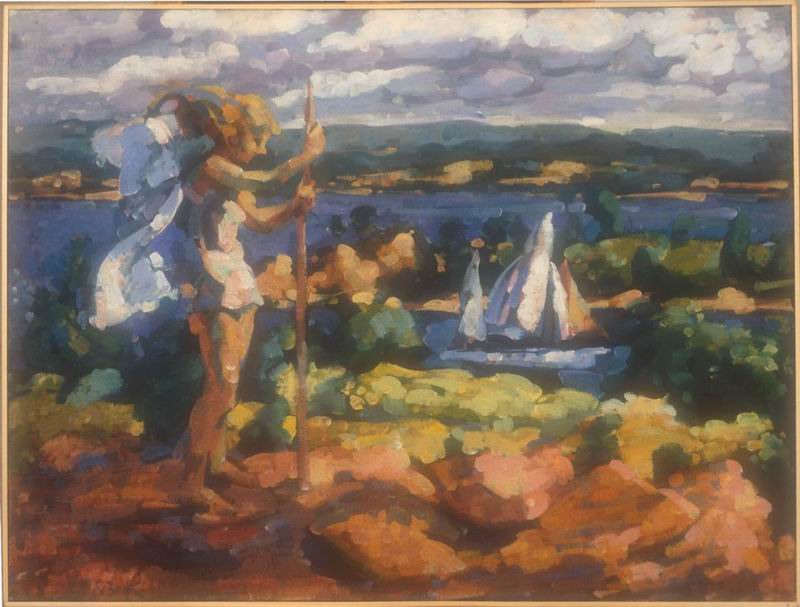The painting, primarily rendered in broad, blobby strokes, depicts an ethereal outdoor scene with a young woman resembling a fairy. On the left side of the image, she stands on a brown, rocky ledge, facing right in a side profile. The fairy-like figure, possibly modeled after Tinkerbell, has dirty blonde hair styled up, and she wears a short, light dress which reveals her legs. She holds a straight staff with both hands and has butterfly-like white wings protruding from her back.

In the distance to the right, a sailboat glides on a blue bay, flanked by verdant green patches suggestive of trees or grass. Further beyond, two rivers converge, leading to more land and distant mountains under a sky adorned with fluffy gray and white clouds. The entire painting is surrounded by a thin, light brownish-yellow border, adding to its charm. The overall color palette includes hues of yellow, brown, white, gray, blue, light blue, green, and light brown, emphasizing its impressionistic and dreamy quality.